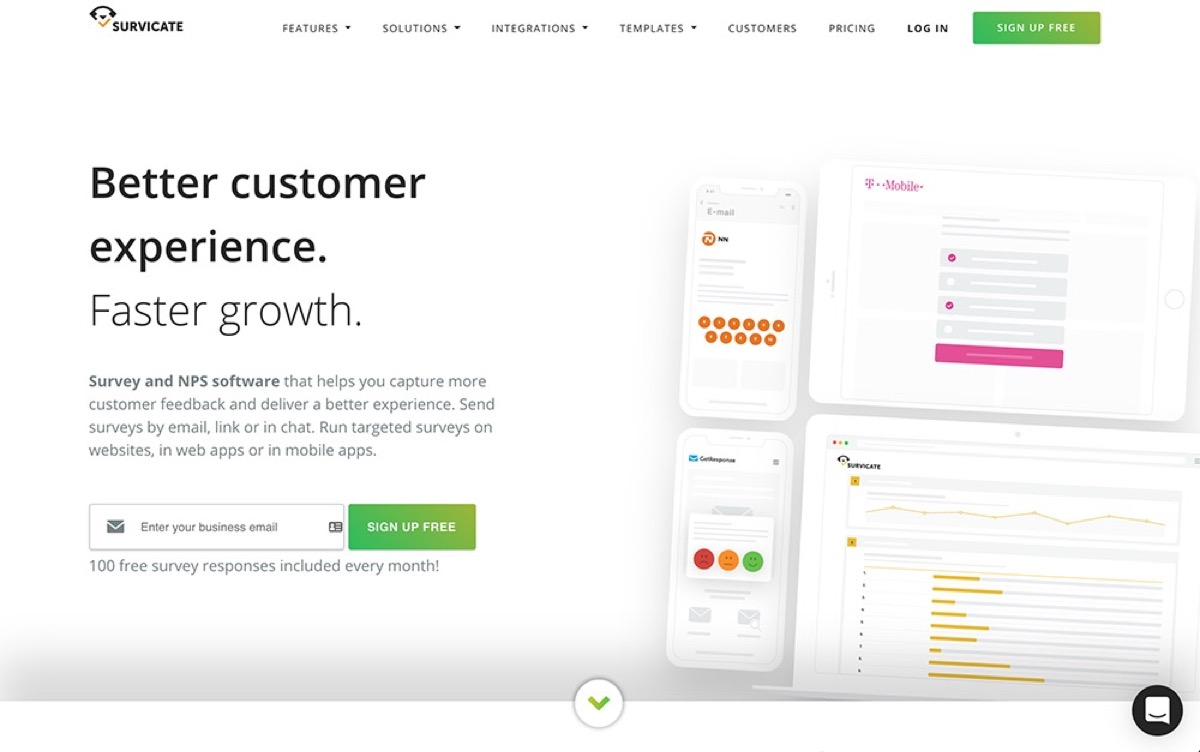The image depicts a web page from the survey website SURVICATE, shown in landscape orientation on an unspecified device. The background is white, with a down arrow centered at the bottom, indicating that the page can be scrolled down.

At the top of the page, there is a horizontal menu with expandable items: "Features," "Solutions," "Integrations," and "Templates." Additional menu items include "Customers," "Pricing," "Login," and a green "SIGN UP FREE" button—all in uppercase, but in small font.

Dominating the left half of the page, bold black text reads "Better Customer Experience. Faster Growth." Note that "Better Customer Experience" is bold, while "Faster Growth" is not. Beneath this, a small-font blurb states: "Survey and NPS Software that helps you capture more customer feedback and deliver a better experience. Send surveys by email, link, or in chat. Run targeted surveys on websites, in web apps, or in mobile apps."

Below this text is another green "SIGN UP FREE" button alongside a text box prompting users to "Enter Your Business Email," featuring an envelope icon. Underneath this prompt, it declares: "100 FREE SURVEY RESPONSES INCLUDED EVERY MONTH!"

The right side of the page is adorned with simple line illustrations in grey with touches of color, depicting two smartphones on the top left and two devices below—likely a tablet and a laptop. The tablet-like device at the top mentions "T-Mobile" in pink, while the laptop-like device at the bottom shows an orange graph and progress bar.

The overall layout is clean and user-friendly, guiding users toward signing up and highlighting the key benefits of the SURVICATE survey platform effectively.